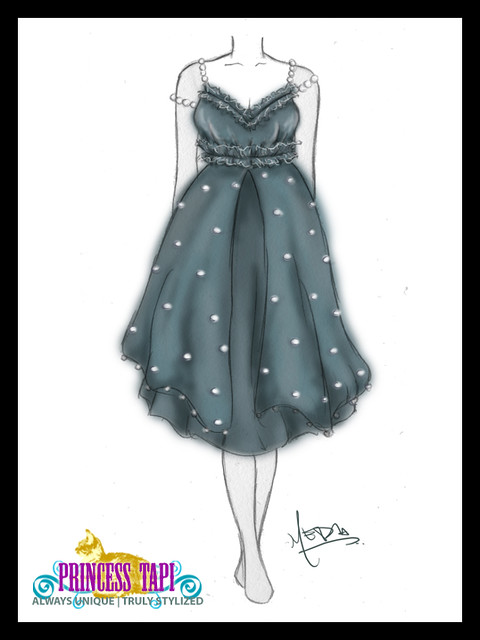The image is a detailed sketch of a knee-length party cocktail dress set against a white background, framed by a dark black border. The dress is black with sheer, greenish-black tones and adorned with delicate white polka dots. The bodice features a V-neckline embellished with lace and ruffles, which also appear just under the bust line. The waist is gathered, accentuating the figure, and the dress flows gracefully down to just below the knees. The straps are intricately designed, resembling beads or pearls, with one set going over the shoulders and another set hanging down. The image excludes details like hands and shoes, focusing solely on the elegance of the dress. In the left-hand corner, a caption reads "Princess Tappy: Always Unique, Truly Stylized."